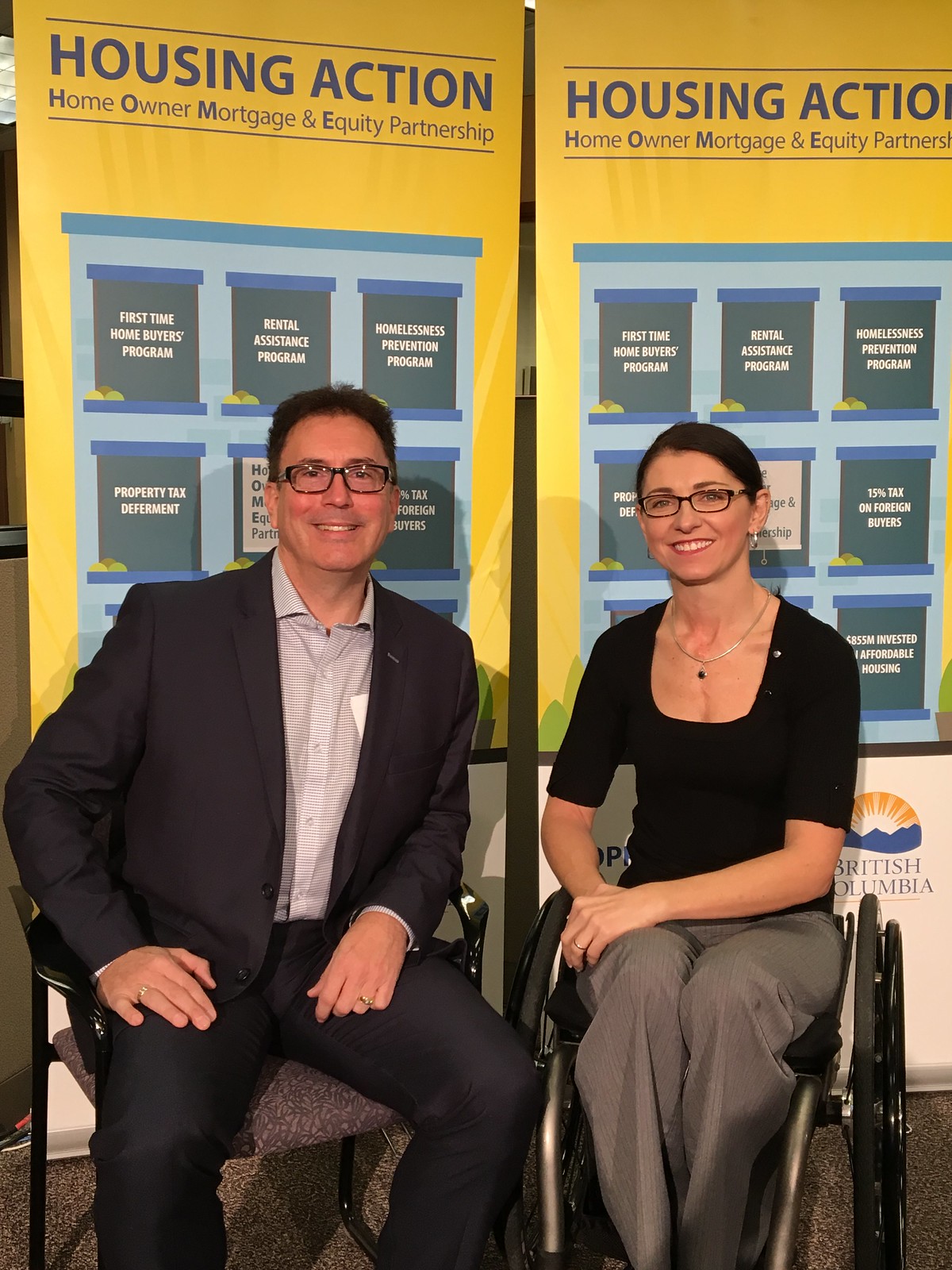The photograph captures a man and a woman sitting next to each other in what appears to be a lobby or conference room with a carpeted floor. Behind them are two identical banners with a yellow background and blue lettering that read "Housing Action: Home Owner Mortgage and Equity Partnership." The banners feature a graphic of a house, with some windows displaying text such as "First-time Buyers Program," "Rental Assistance," "Homelessness Preventative Program," "Property Tax Department," and "15% Tax on Foreign Buyers," although some of the windows are obscured by the individuals' bodies in the foreground.

The man, seated on the left in a gray cushioned metal chair, is wearing black dress pants, a black business coat that is unbuttoned, and a red-and-white striped shirt with the top button undone. He also has black-framed glasses. The woman to his right is in a black wheelchair, wearing black-framed glasses, a black jacket over a checkered white shirt, and gray pants. The setting, marked by the indoor atmosphere and distinct carpet pattern, suggests a professional or formal event related to housing or real estate initiatives.